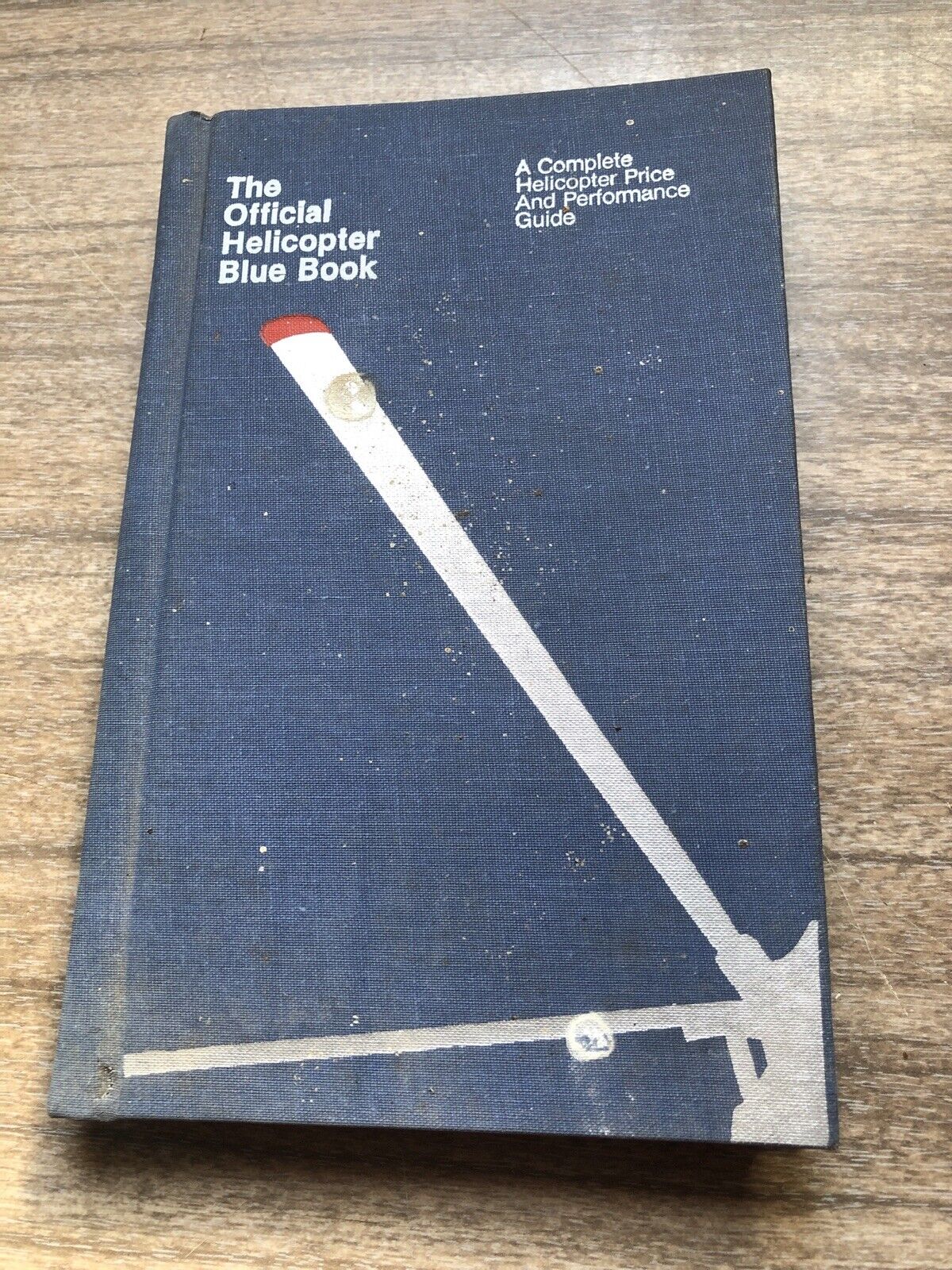The photograph captures an old, dark blue canvas-bound book titled "The Official Helicopter Blue Book – A Complete Helicopter Price and Performance Guide," resting on a horizontally grained wooden table. The table's wood grain varies from light to dark brown-grey shades. The book exhibits signs of age with visible dirt, dust, and white markings, particularly concentrated towards the bottom. The white, faded font of the title is prominently displayed at the top, with "The Official Helicopter Blue Book" in larger letters and "A Complete Helicopter Price and Performance Guide" in slightly smaller text. Dominating the cover is a minimalistic white silhouette of a helicopter's rotors, with the visible portion of the helicopter located in the bottom right corner. The rotors extend diagonally across the book, and one of the larger rotor blades features a red tip.